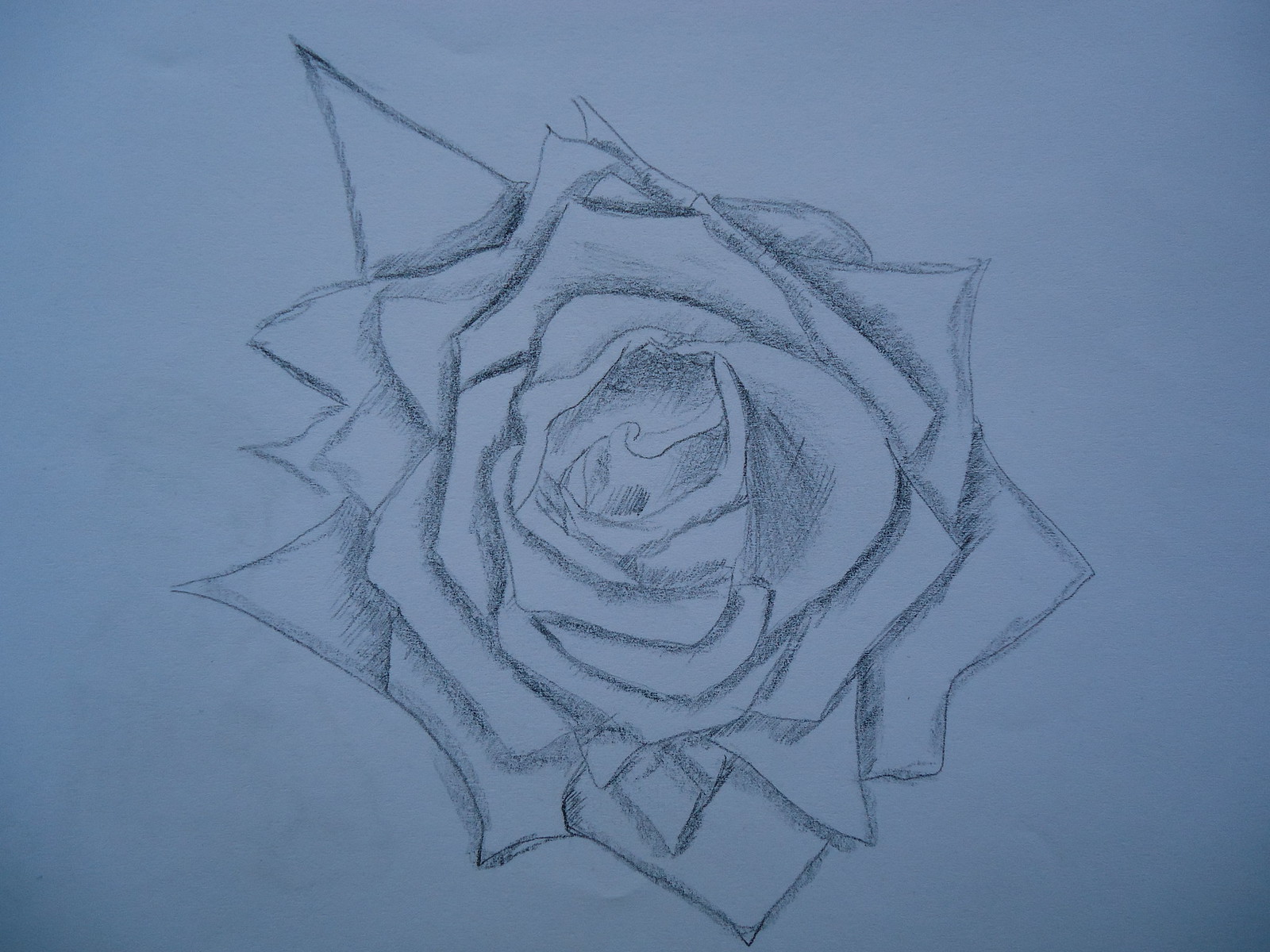The photograph captures a detailed pencil drawing of a fully bloomed rose, viewed from above. The rose is depicted on a piece of off-white paper with a subtle bluish tint. The intricate sketch showcases multiple overlapping petals that extend outward, becoming more jagged and triangular towards the edges. Among the petals, there are larger triangular shapes emerging from the upper left corner and the lower center-left, likely representing leaves, although they remain uncolored like the rest of the drawing. All elements are rendered with a clear line outline and some shading between the petals, giving the sketch a realistic yet stylistic appearance.